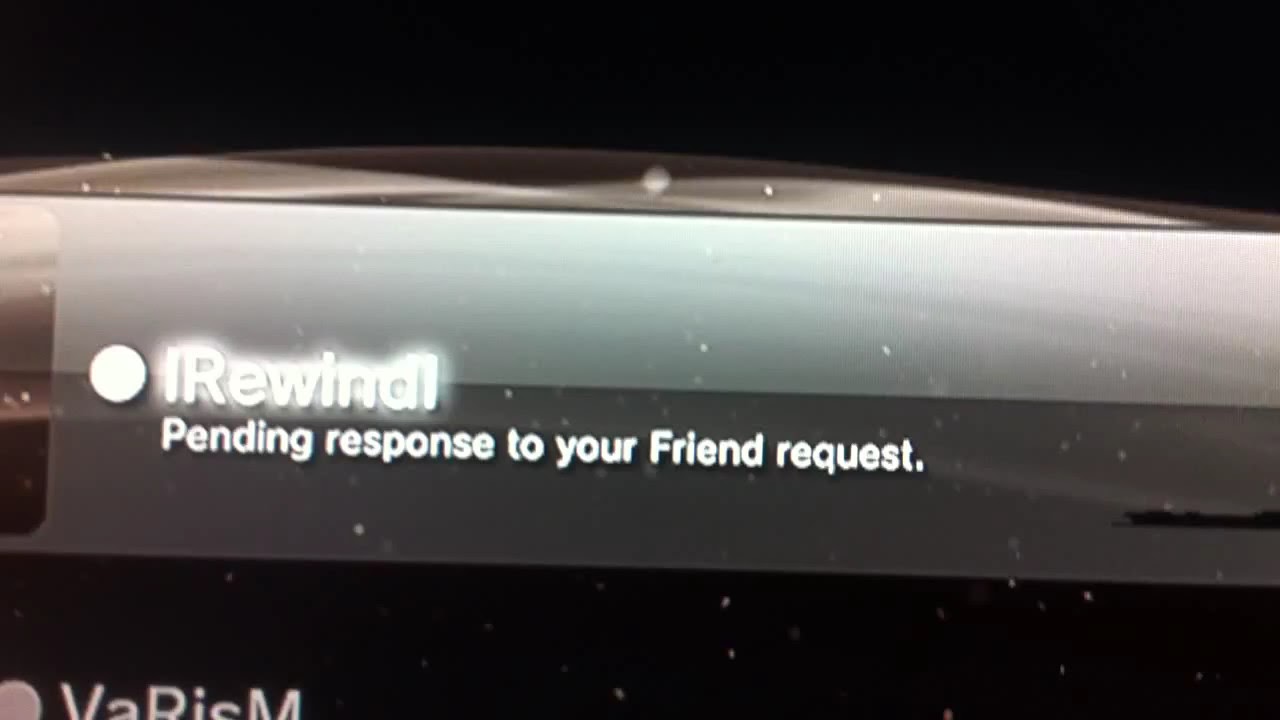The image appears to be a photo taken of a TV screen displaying a notification. The background is predominantly dark, with black areas at the top and bottom where text is partially cut off. In the middle, there's a wide silver or light gray line, overlayed by a notification card in a light green gloss that includes white text. A circle with white dots is featured prominently, possibly indicating focus on the alert.

The notification reads "I Rewind" with horizontal lines flanking the text, and beneath it, in a smaller font, it states "Pending response to your friend request." The notification card also displays a mix of uppercase and lowercase letters, spelling out "VARISM" in white text toward the bottom, though it's partially truncated. The text is aligned with dark wavy lines and other white dots, adding to the screen's detailed visual complexity.